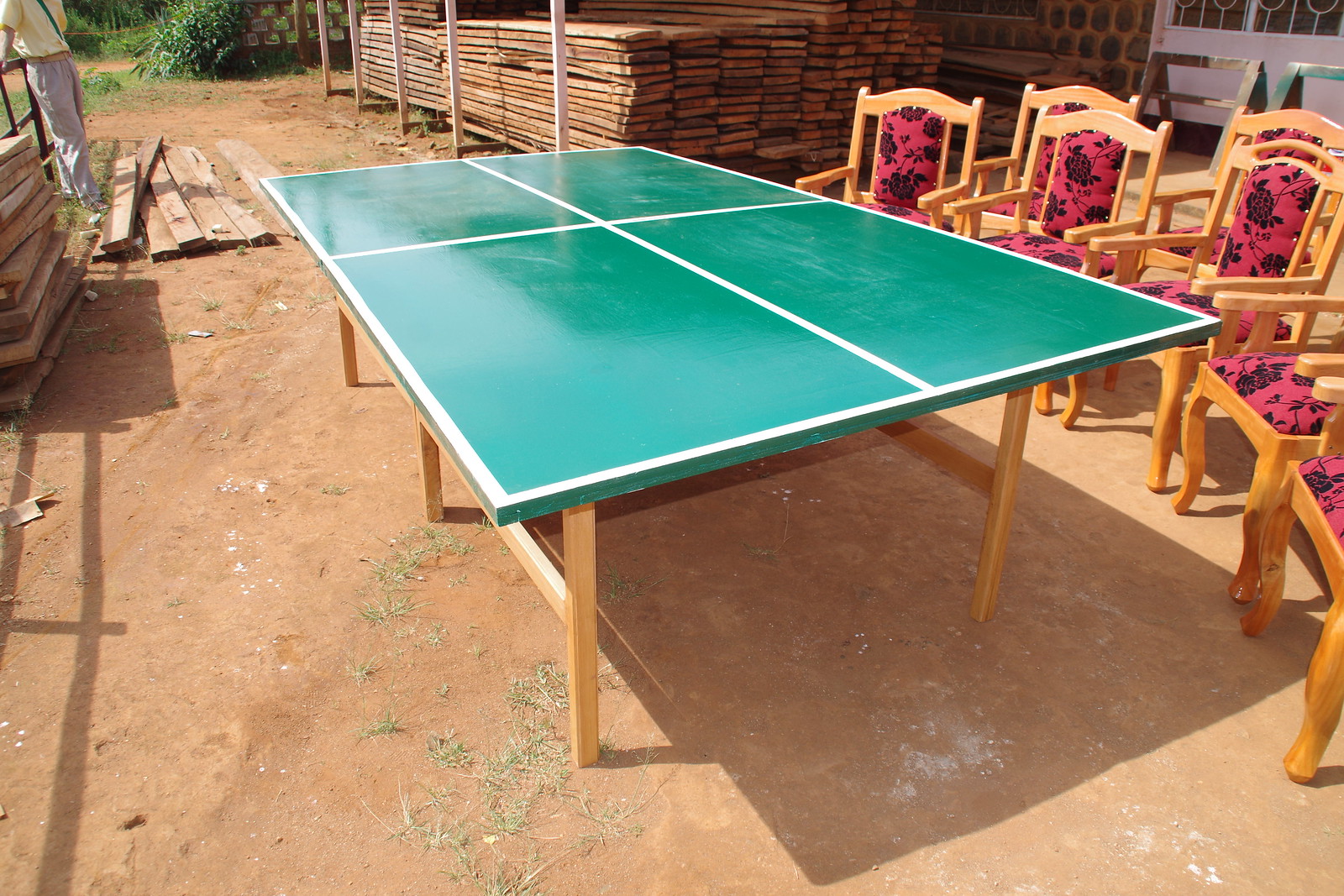The photograph captures an outdoor scene, possibly at a woodworker's workshop, evident from the stacks of lumber in the background near what appears to be a storage garage with visible garage doors to the right. The ground is covered in red dirt. Central to the image is a long, rectangular ping-pong table, painted green with a white border and two intersecting white lines forming a smaller rectangle design on the table's surface. Surrounding the table on the right side are several (at least seven) light wood upholstered chairs featuring red fabric with black rose designs. In the background, to the left, stands a man in khaki pants and a yellow shirt, partially visible from the shoulders down.